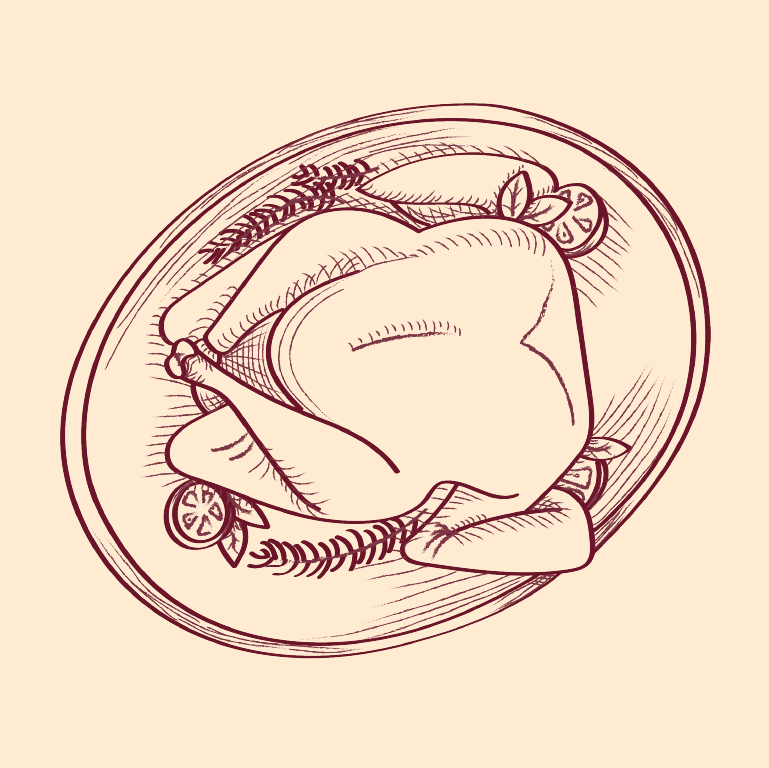The image portrays a minimalist line drawing of a cooked turkey resting on a thick, rounded platter, which is set against a pink or cream background. The platter is depicted at an angle, tilting from a lower left to a higher right, with the turkey positioned almost horizontally across it. The turkey's legs are drawn towards the left, while the area where the head would be is oriented to the right. Surrounding the turkey are sprigs of rosemary—one at the bottom, one on the left side, and one on the right side of the plate—drawn simply with lines and half circles. Additional garnishes that resemble lemon halves, although some suggest they look like tomatoes, are scattered around the turkey, placed under its wings and the left drumstick. The drawing employs cross-hatching to add depth and dimension, particularly notable on the turkey's breast and belly. Despite some peculiar details, such as a line on the breast that appears almost like stitching, the simplicity and identifiable features of the drawing make it clear and well-executed.